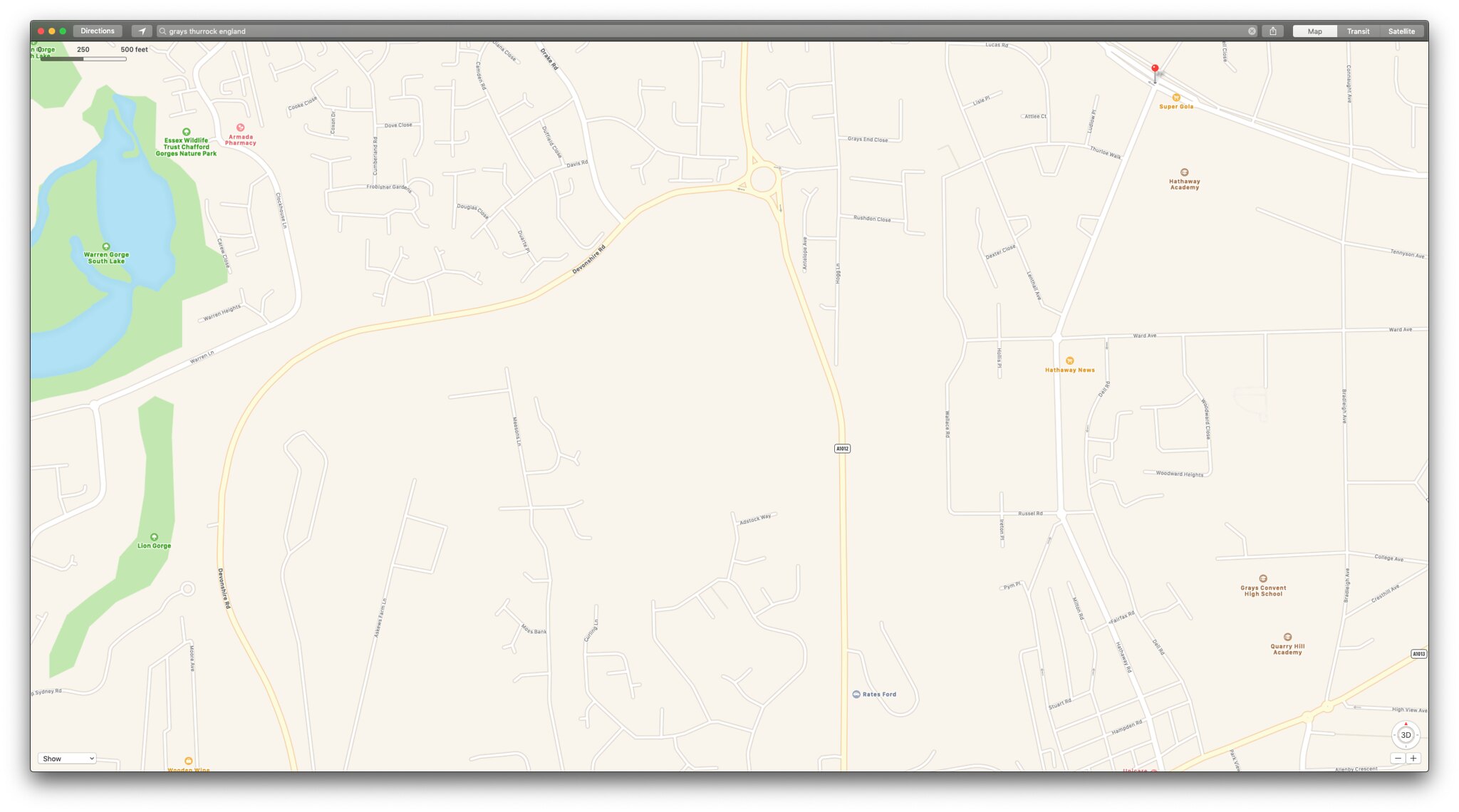The image is a screenshot of a computer screen displaying a digital map interface, typically used for navigation or seeking directions. The interface features a dark gray strip at the top, which houses three colored circles on the left: red, yellow, and green, likely representing window control buttons. Beneath this strip, there is a lighter gray box labeled "Directions." Adjacent to it on the right is a smaller rectangular box with an arrow pointing up to the right, suggesting an option to minimize or expand. Following this, a search bar adorned with a magnifying glass icon contains the text "Grays, Thurrock, England."

The main map area displays a pale brown background with labeled streets, accented by green areas indicating parks and blue regions representing bodies of water. Points of interest, such as specific stores, are marked in red, including the "Armada Pharmacy." Additionally, the right side of the map highlights two schools in brown: "Grays Convent High School" and "Quarry Hill Academy." This detailed and colorful depiction aids users in visually navigating and locating key places within Grays, Thurrock, England.